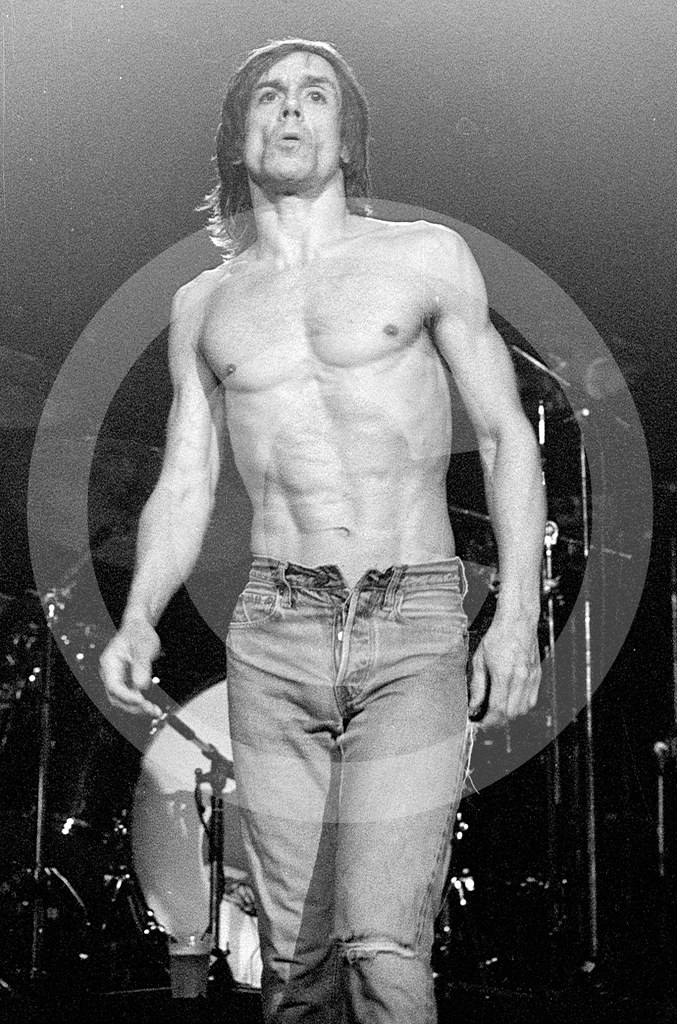In this striking black-and-white image, a shirtless, light-skinned male singer with medium-length dark hair cascading to his shoulders stands in a confident pose. His lean, muscular frame is accentuated by the contrast of his blue jeans, which are provocatively unbuttoned at the waist and feature a prominent rip at the left knee. His arms hang naturally at his sides, contributing to the raw, unpolished feel of the scene.

The backdrop suggests a music stage, with various microphones and musical instruments, including a partially obscured drum set with a visible cymbal. This setting is enhanced by a translucent white semicircle resting on his left side, from his hip to just below his knee, adding a subtle artistic touch to the composition. A gradient of grays, whites, and blacks creates a moody atmosphere, completing the image’s gritty, performative aesthetic. At his feet lies a glass of beer, crowned with a small layer of foam, grounding the scene in a moment of casual, candid reality.